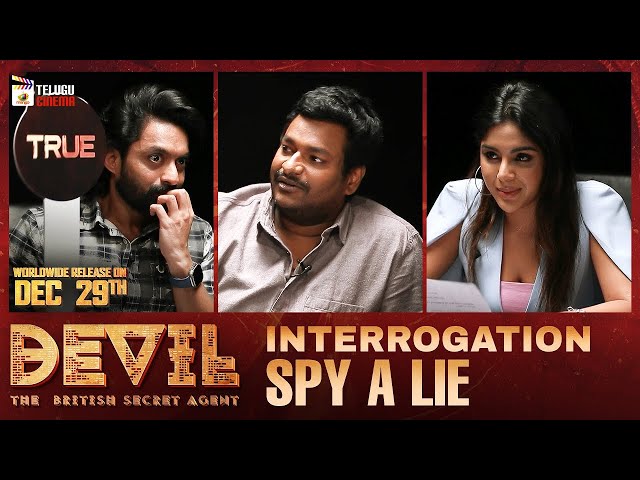The image is an advertisement for a movie or TV show, presented in a wide vertical rectangular format with a black background. Across the center, divided into three vertical sections by dark red trim, are portraits of three individuals, all likely of Indian or Middle Eastern descent, each with brown skin and black hair.

On the far left is a man with black hair, a full black beard, and a mustache. He is wearing a green and white plaid button-down shirt and has his hand over his mouth, facing towards the right. To his right is another man, slightly older, with black hair and a black mustache. He is wearing a gray button-down shirt and is leaning towards the right, his face turned towards the left.

The rightmost section features a young woman in her 20s. She has long, straight black hair parted in the middle, extending just over her chest. She has brown eyes, brown skin, and a round earring on her left ear. She is dressed in a light blue cape over her shoulders and a pink shirt.

Above the portraits, there is an illustration of a clapperboard and the text "Telugu Cinema." Beneath the portraits, prominently displayed text reads "Worldwide Release on December 29th." Additional text in symbol-style letters says "Devil, the British Secret Agent," and to its right, "Interrogation, Spy a Lie."